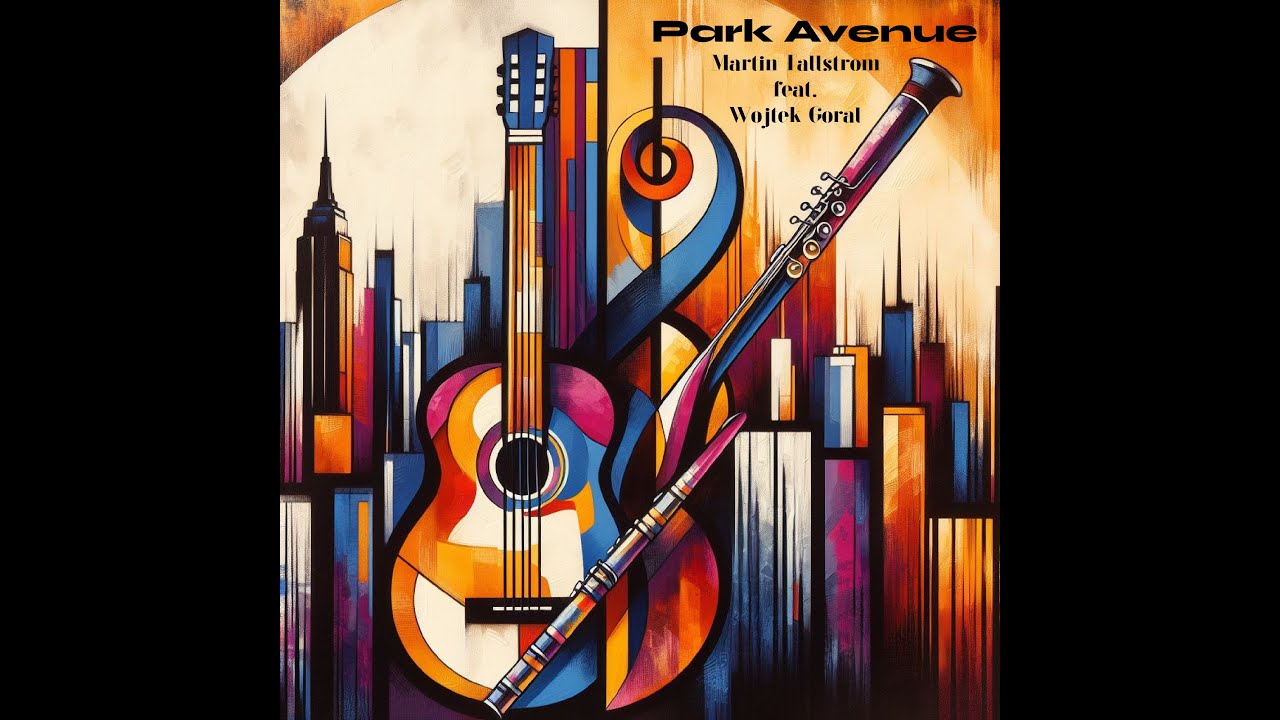The image features a vibrant and abstract graphic design, likely serving as an album cover or advertisement for a music event. Set against a black background, the square-shaped composition is dominated by colorful, cubist-inspired artwork reminiscent of Picasso. In the top right corner, black text reads "Park Avenue, Martin Tillstrom featuring Wojtek Goral." The central theme of the painting showcases a cityscape composed of tall, slender buildings in a mosaic of colors: black, red, brown, blue, yellow, white, and purple. Emerging from this bustling skyline are various musical instruments, including a guitar, a horn, and a flute, all depicted in a multicolor palette. The overall design is dynamic, with intricate geometry and an explosion of hues such as orange, yellow, blue, and pink, lending a lively and artistic flair to the promotional piece.